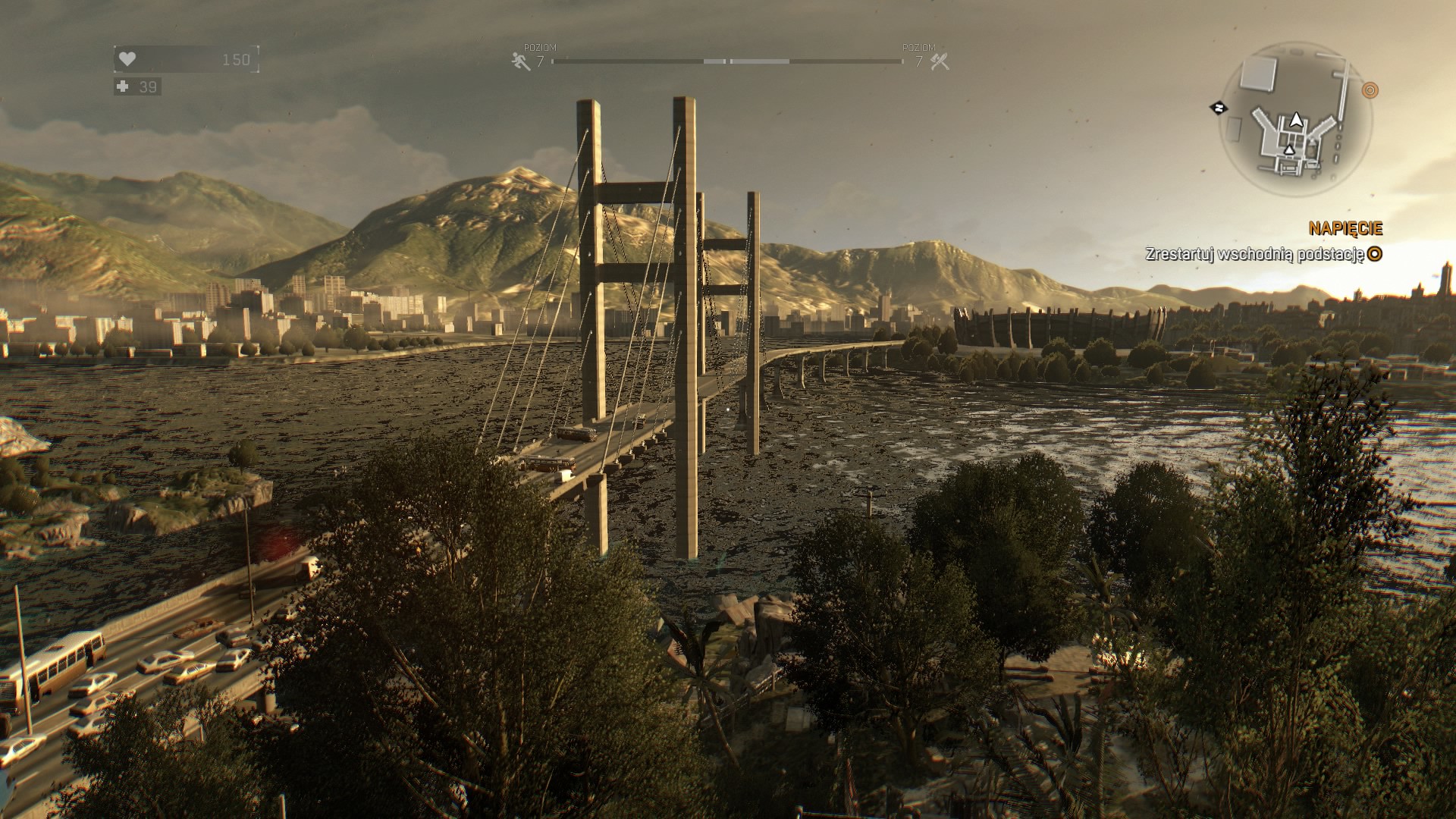This is a highly detailed screenshot from a video game, featuring a digitally rendered landscape that closely resembles the Golden Gate Bridge in San Francisco. The bridge spans from the left side of the image towards the middle, making a right-hand turn above a watery expanse. Intricately designed, the bridge displays its iconic giant cables in taupe, brown, gray, and black hues, and supports various vehicles including a distinctively colored bus with a white top and burnt orange bottom, plus numerous smaller cars.

In the foreground, on the left side, a gaming HUD displays a dark-to-light gradient rectangle with a white heart icon and the number 150, indicating the player’s health status. Below it, another shorter rectangle features a white plus symbol next to the number 39, possibly adding health points. Additionally, a long skinny bar in the center, flanked by an X on the right and a microphone with a line through it on the left, hints at more game controls. A circle at the top right featuring a box-like icon and the text "H-A-P-I-E-C-I-E" adds to the game’s interface elements.

Background details enhance the scene's realism with verdant green and white mountains, variously shaped and sized white skyscrapers, and dense clouds in a gloomy, gray sky. Brush and trees frame the bridge on the right side, contrasting with housing and more mountains to the left, creating a richly textured and immersive visual environment.